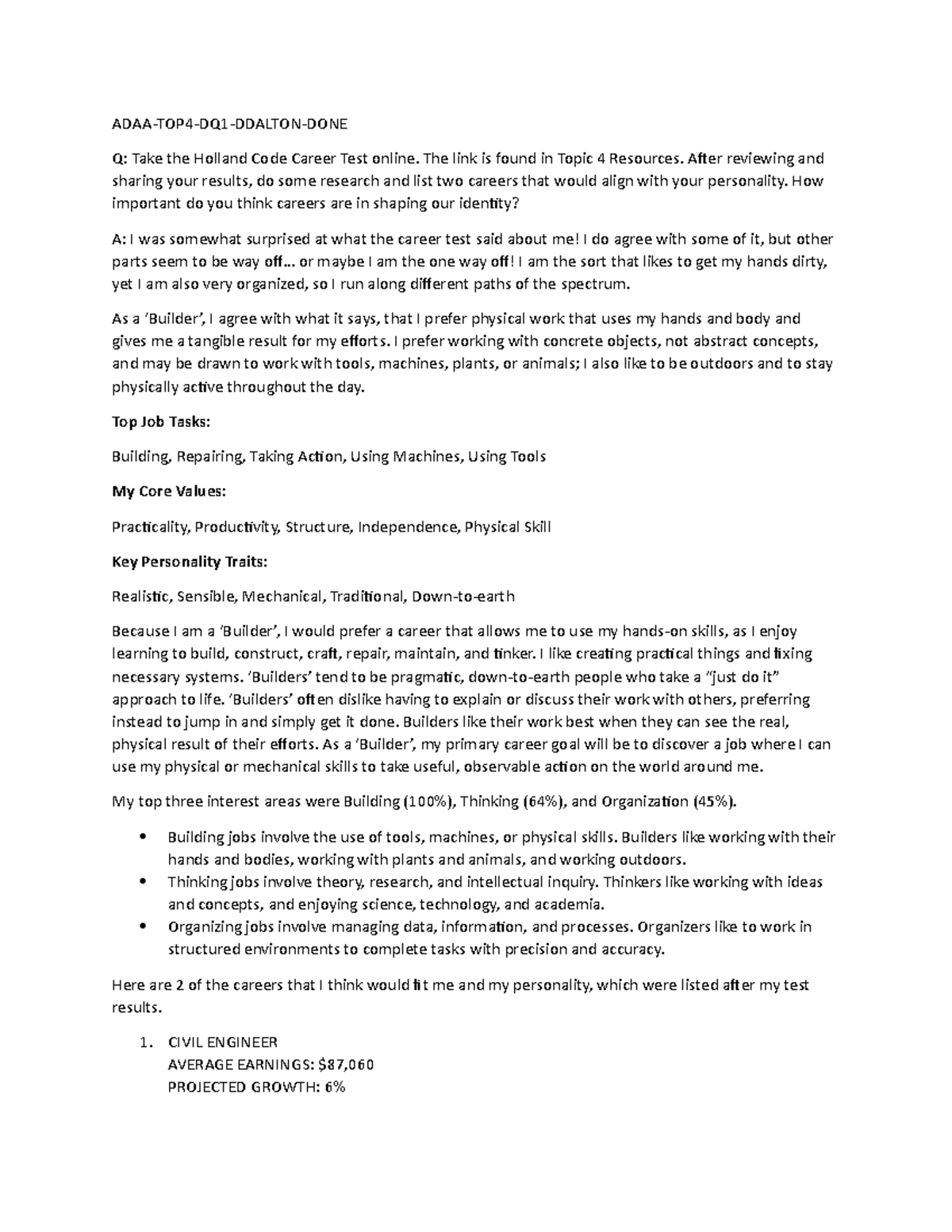The image showcases several paragraphs of text discussing job recommendations aligned with personal traits and core values. One particular profile highlighted is of a person who enjoys physical outdoor work, such as building with concrete blocks, handling machinery, and working with tools and plants. The job recommendation site confirmed that this individual's preferences matched with top careers in building, repairing, taking action, and utilizing machines and tools. Core values underscored in these recommendations include practicality, productivity, structure, independence, and physical skills. Key personality traits identified were realistic, sensible, mechanical, traditional, and down-to-earth. The text elaborates on how interests in building, logical thinking, and organization harmonize, providing a detailed breakdown of suitable careers for someone inclined towards hands-on, physical tasks rather than purely intellectual challenges.